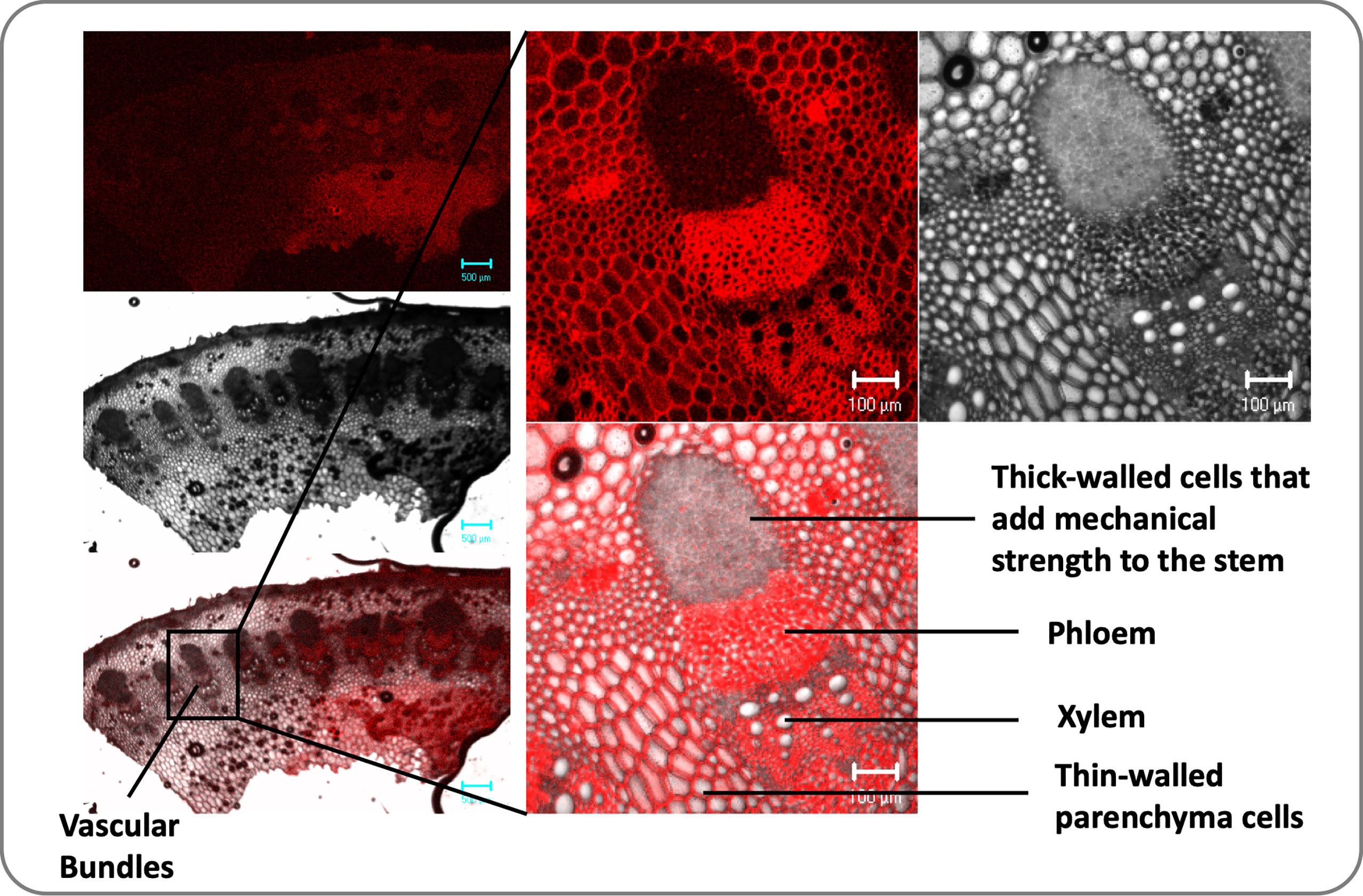The image is a detailed collage of seven microscopic photographs, each depicting various cellular structures of the human body at a highly magnified level. The images are primarily in shades of red and grayscale, creating a vivid and somewhat eerie contrast. 

On the left side, three images are stacked vertically. The top-left image is dark with red highlights, reminiscent of a spooky underwater scene. Below it, a series of cross-sections of vascular bundles is shown, labeled with descriptive text and black lines for zooming in on specific areas. An even more magnified image of these vascular bundles is displayed beneath, showcasing different hues to highlight cellular details. 

To the right of this column, two more images are stacked vertically. The top one continues the series of magnified vascular bundles, while the bottom one features an even closer examination of cellular structures, showing thick-walled cells that contribute to mechanical strength, phloem, xylem, and thin-walled parenchyma cells. Each image includes measurement scales, often reading 100 micrometers, to indicate the level of magnification. 

In the upper right corner, there is a singular image accompanied by blank white space with text identifying various cell parts and their functions. This arrangement allows for a comprehensive view of dense, circular, cell-like structures, emphasizing the intricate details of the vascular bundles and their role within the stem.